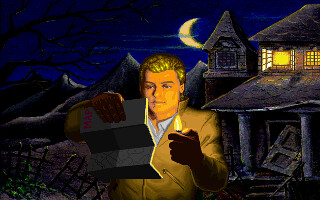In this computer-generated, possibly video game screen capture, a young, blonde man in a tan trench coat and red gloves stands outside at night, holding an unfolded map in his right hand and a lighter in his left to illuminate it. The scene is set in front of an abandoned, potentially haunted house with broken-down, rickety fencing. The house features an eerie, busted front door, cobwebs seemingly streaming from the roof, and lit windows on the second floor, one of which is open. Behind him, a dark sky with a crescent moon and thin clouds looms over pointy mountains. There's also a scraggly, leafless tree adding to the desolate atmosphere. The image, showing clear pixelation, hints at being a point-and-click hidden-object game.